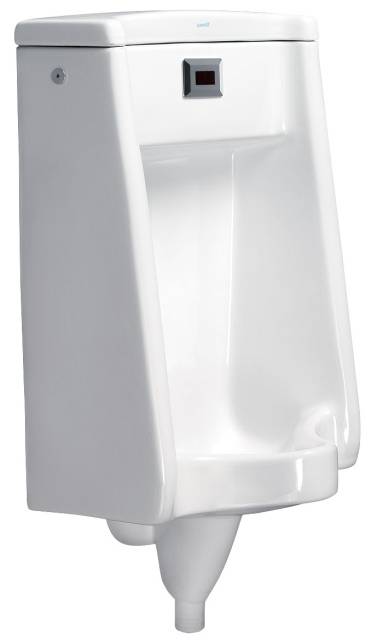This particular image features a white porcelain urinal, distinctly set against an all-white background, giving it the appearance of floating. The urinal resembles typical toilet fixtures, with a lid on top similar to the ones found on the back of toilets, beneath which one would expect to find the water and ball flusher mechanism. A small gray square is prominently positioned at the front, likely serving as the flusher. On the left side, there's a noticeable metal circle, probably intended to secure the urinal to a wall. Additionally, there is piping at the bottom that should connect to the plumbing, though in this image, it appears unattached. The urinal is detailed with an indented section, possibly designed for ease of use. There is also some tiny, illegible text at the top, potentially indicating the manufacturer's name. The image captures the urinal from an angle where the left side is shaded while the front is illuminated, highlighting these various features.